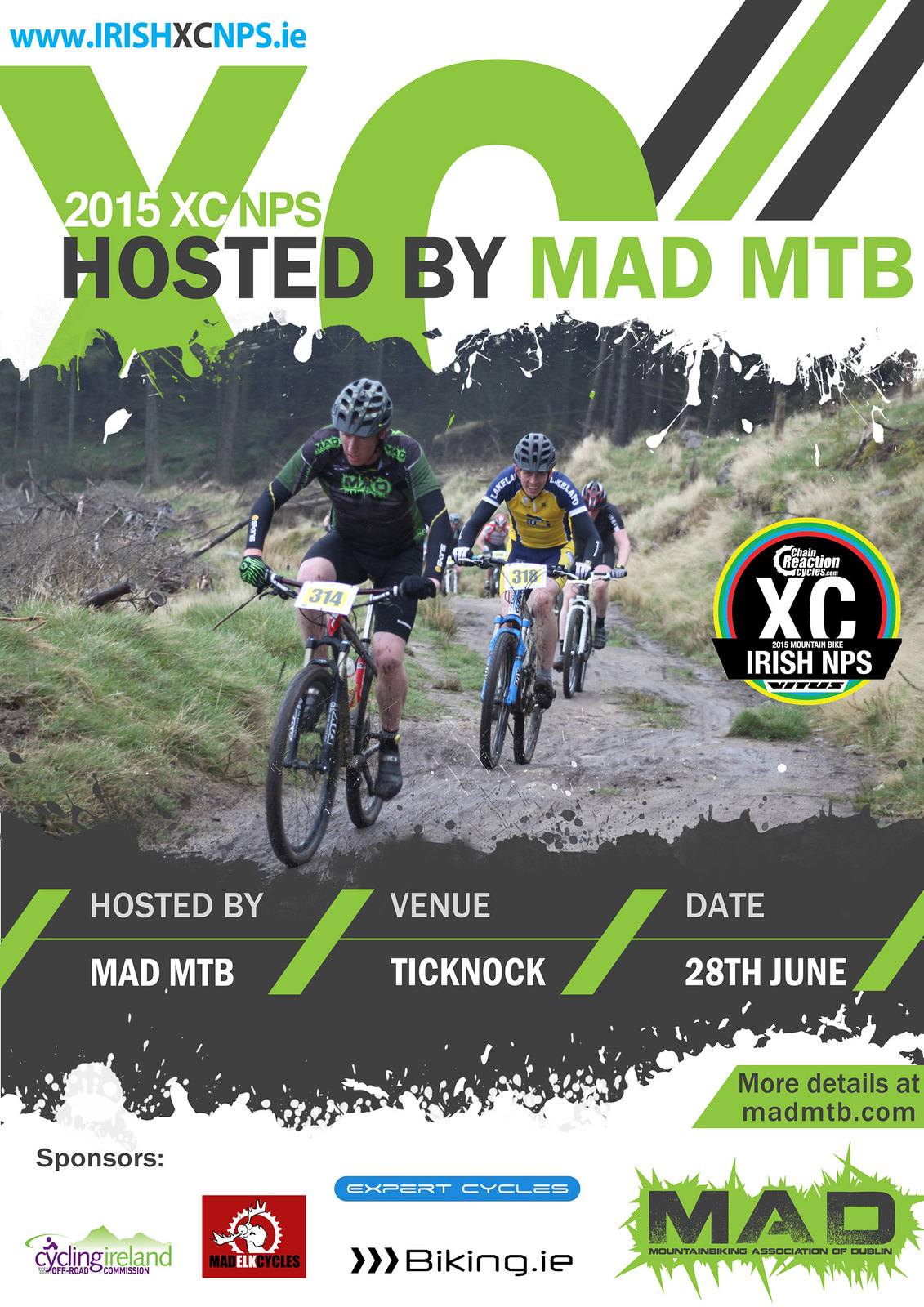This promotional poster for the 2015 XCNPS event, hosted by MadMTB, features a combination of detailed visual and textual components. At the top of the poster, the web address www.irishxcnps.ie is highlighted in blue, with “XC” appearing in black. Immediately below, a large green "XC" is prominently displayed, overlaid with “2015 XCNPS” in white and green text. A striking design element includes diagonal stripes running from the bottom left to the top right, alternating between black, white, and green, culminating in the red text of "hosted by Mad MTB."

The central photograph showcases a dynamic image of bicyclists donned in colorful sports uniforms, numbered 314 and 318, riding on a dirt trail through a grassy area flanked by what looks like orchard trees. All riders are wearing helmets. Additionally, a prominent black circle with concentric rings in red, blue, green, and yellow surrounds the text "Chain Reaction XC Irish NPS."

Further details at the bottom of the poster provide logistical information: “Hosted by Mad MTB, Venue: Ticknock, Date: 28th of June.” The footer, set against a white background, lists the event’s sponsors, including Cycling Ireland, Expert Cycles, Mad Mountain Association of Dublin, among others, with a green strip indicating where more details can be found at madmtb.com.